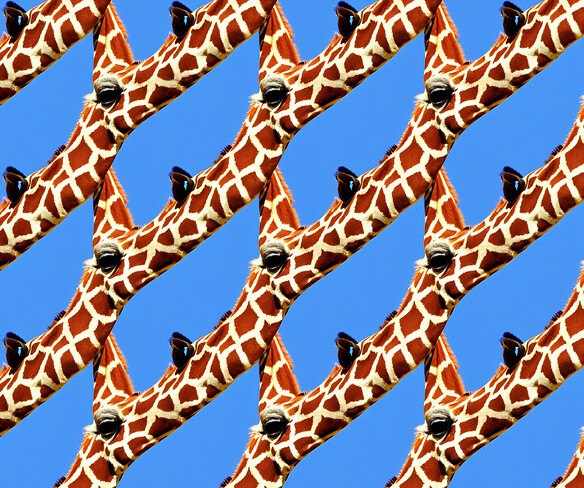This image features a highly detailed and unique composite design of giraffe heads and necks melded together. Set against a vibrant electric blue sky background, the giraffes are arranged in six diagonal rows, each one seamlessly fused to the next, creating a continuous and intricate pattern. The heads, eyes, and ears of the giraffes are prominent, each possessing identical brown and white markings with black accents, including dark eyes and pointed ears. The necks are merged in such a manner that it is challenging to distinguish where one giraffe begins and another ends, producing an almost fence-like structure. The detailed brown patchwork on white with black highlights adds to the visually striking and peculiar aesthetic of the image. This intriguing artwork could be an altered photograph, a drawing, or even a poster with a textile-like appearance due to its detailed and repeated pattern elements.